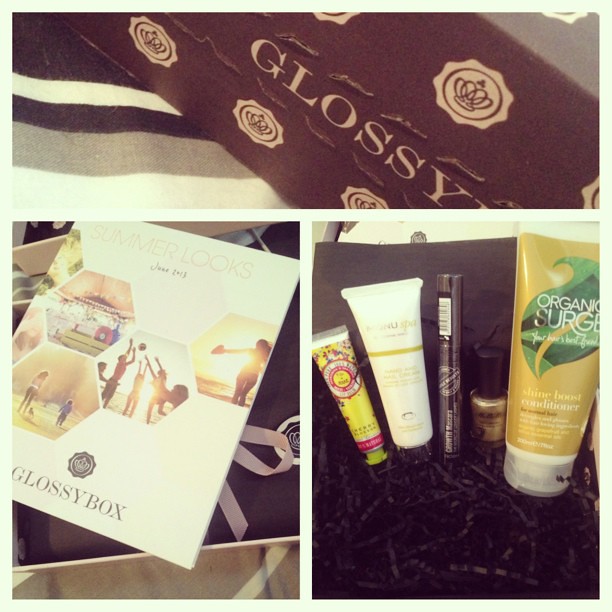The image is a collage of three distinct photos. At the top, there is a photograph of a stylishly designed brown box labeled "Glossy" in tan writing, decorated with circular logos featuring crowns. Below this, the collage splits into two side-by-side photos. The left photo showcases an open box with a magazine draped across it, titled "Summer Looks June 2013 Glossy Box." The magazine cover is decorated with a collection of hexagonal images depicting people enjoying summer activities like beach volleyball and walking outdoors. On the right, the final photo displays a lineup of various cosmetic products such as skin lotions, nail polish, and conditioners. Notable items include a tan bottle of "Organic Surge Shine Boost Conditioner," a green and pink lotion, a white product possibly makeup, and a gold-colored nail polish. All these products are presumably part of the "Glossy Box" subscription seen in the magazine.